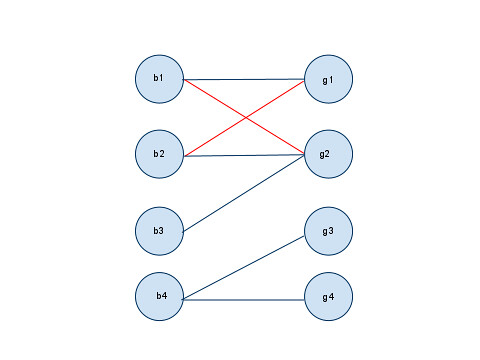A minimalist graphic illustration on a plain white background features two distinct columns of light blue circles, each outlined in a darker shade of blue. The left column consists of circles labeled B1, B2, B3, and B4, while the right column includes circles marked G1, G2, G3, and G4. Thin lines, some red and others blue, connect specific circles, creating a network-like pattern. 

- B4 is connected to both G4 and G3.
- B3 is linked to G2.
- G2 has multiple connections: B3, B2, and B1.
- B1 is connected to G1 and G2.
- G1 is connected to B2 as well.

Among these connections, red lines distinctly highlight the connections between B1 and G2, and G1 and B2. The overall graphic is simple with thin lines and small, thin text, hinting at a technical or conceptual diagram without immediately apparent context or purpose.